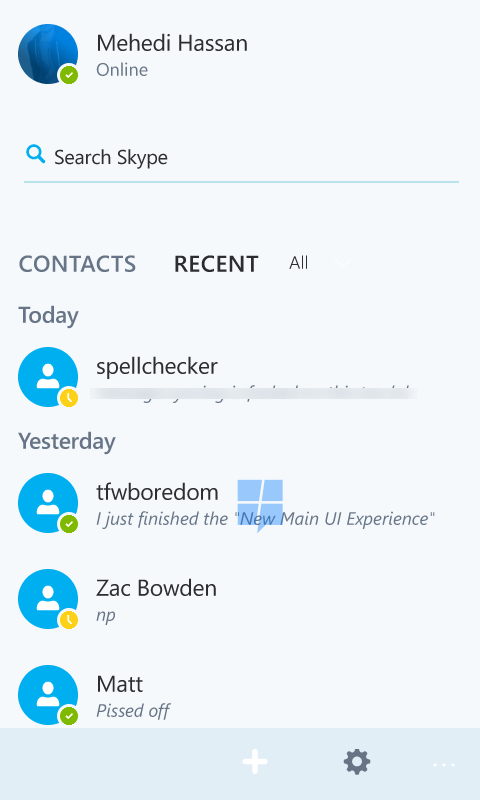On the interface, a vibrant blue circle and a green checkmark signal that Mehdi Hassan is online, standing out against the grey background of the Skype search page. The screen shows various UI elements: a section marked "Recent" highlighting conversations from today which includes a blue circle indicating an unread message. Yesterday's messages flag more blue circles, one labeled “tfw boredom” and another highlighting the completion of the new main UI experience. Two prominent blue circles hold messages from Zack Bowden and Matt, with the latter indicating a sentiment of being "pissed off." 

In the lower interface, a grey rectangle houses a white plus sign, a grey gear icon, and white dots, perhaps denoting settings or additional options. The reverse side of the page is marked by Microsoft's speech recognition feature, showing Mehdi Hassan's online status again. A blue element from the previous day and indications from a spell checker appear before the screen transitions to an all-grey section, concealing details with the note "tfw boredom" surfaced amidst the hidden sections.